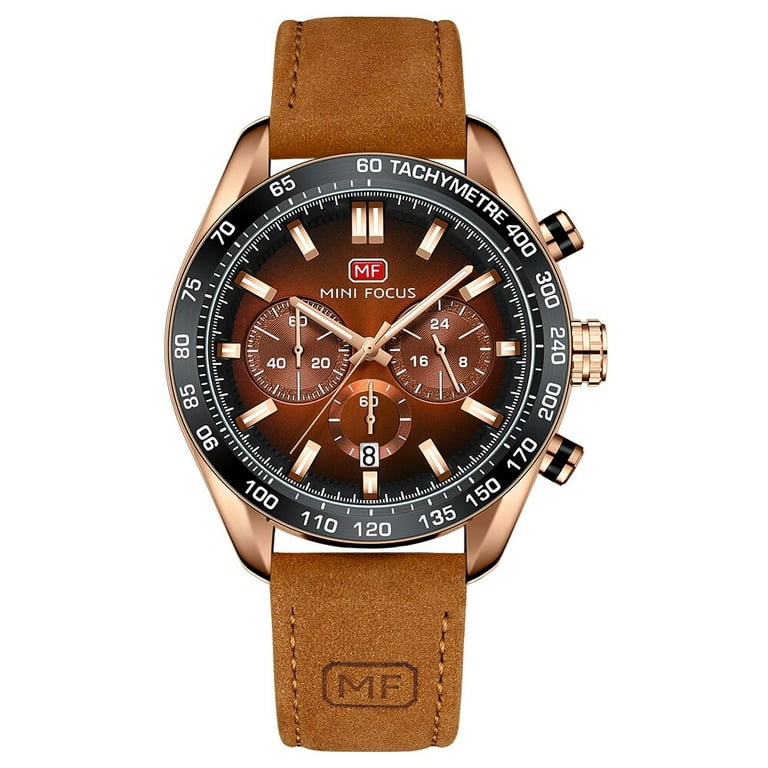The image features an elegant wristwatch with a light brown leather strap, which showcases detailed stitching and a rectangular spot engraved with the brand name "MF" (Mini Focus). The watch face is encircled by a black bezel marked with the text "Tachymeter" and a scale ranging from 60 to 400. The main dial, resplendent in a rich bronze to light gold color, has hour and minute hands paired with 12 large dashes for easy time reading. The text "Mini Focus" and a small red rectangle adorn the center. Additionally, the watch displays three sub-dials: one with the numbers 20, 40, and 60; another marked with 8, 16, and 24; and a third featuring just 60, each with their own small dial. The watch includes three gold-accented buttons on the side, adding to its sophisticated design. Text on the side reads “Apache Leader,” further emphasizing the watch’s premium detailing.